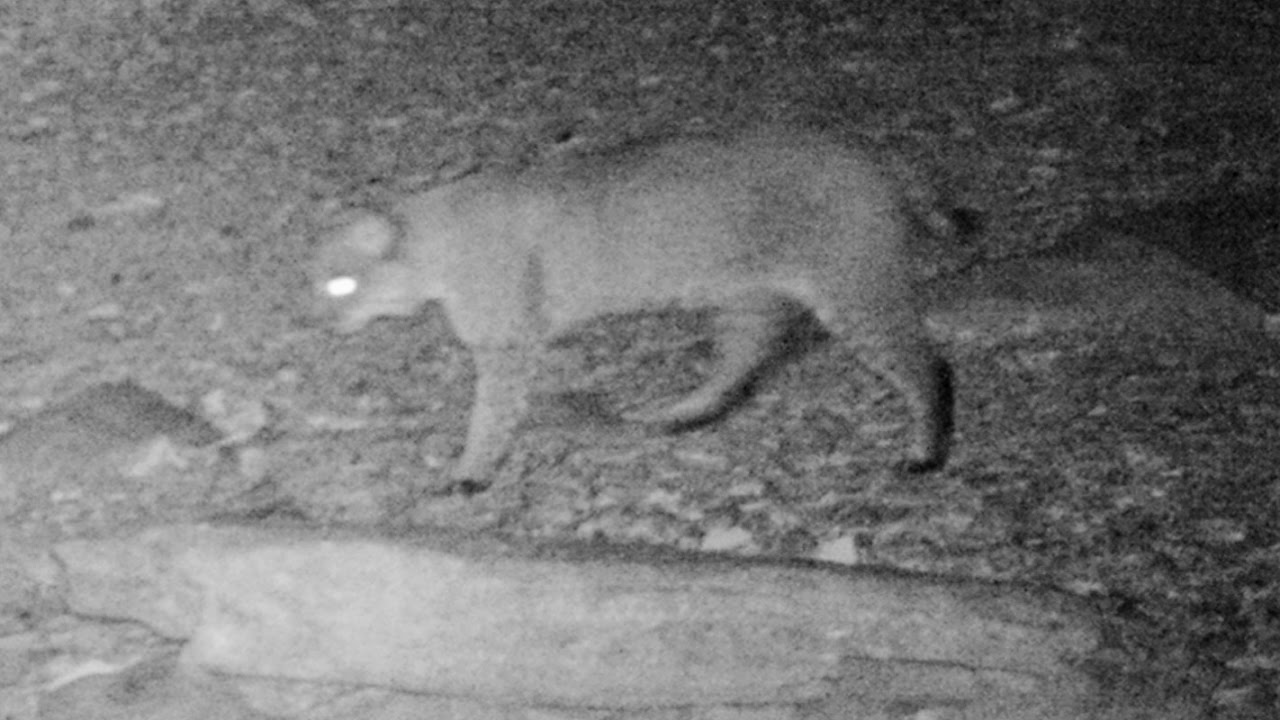This black and white nocturnal photograph features a grainy and gritty aesthetic, typical of surveillance or trail camera footage. Taken at night with a flash or infrared light, the image captures a side view of a feline, most likely a mountain lion or possibly a wild cat, walking cautiously next to a log on the ground. The feline, which seems lighter in color with potential darker markings around its paws, tail tip, and subtle striping, displays a brilliantly reflective, glowing eye—a hallmark of night photography. The scene unfolds in an outdoor setting, likely caught by a trail camera, giving a realistic and slightly eerie quality to the image.